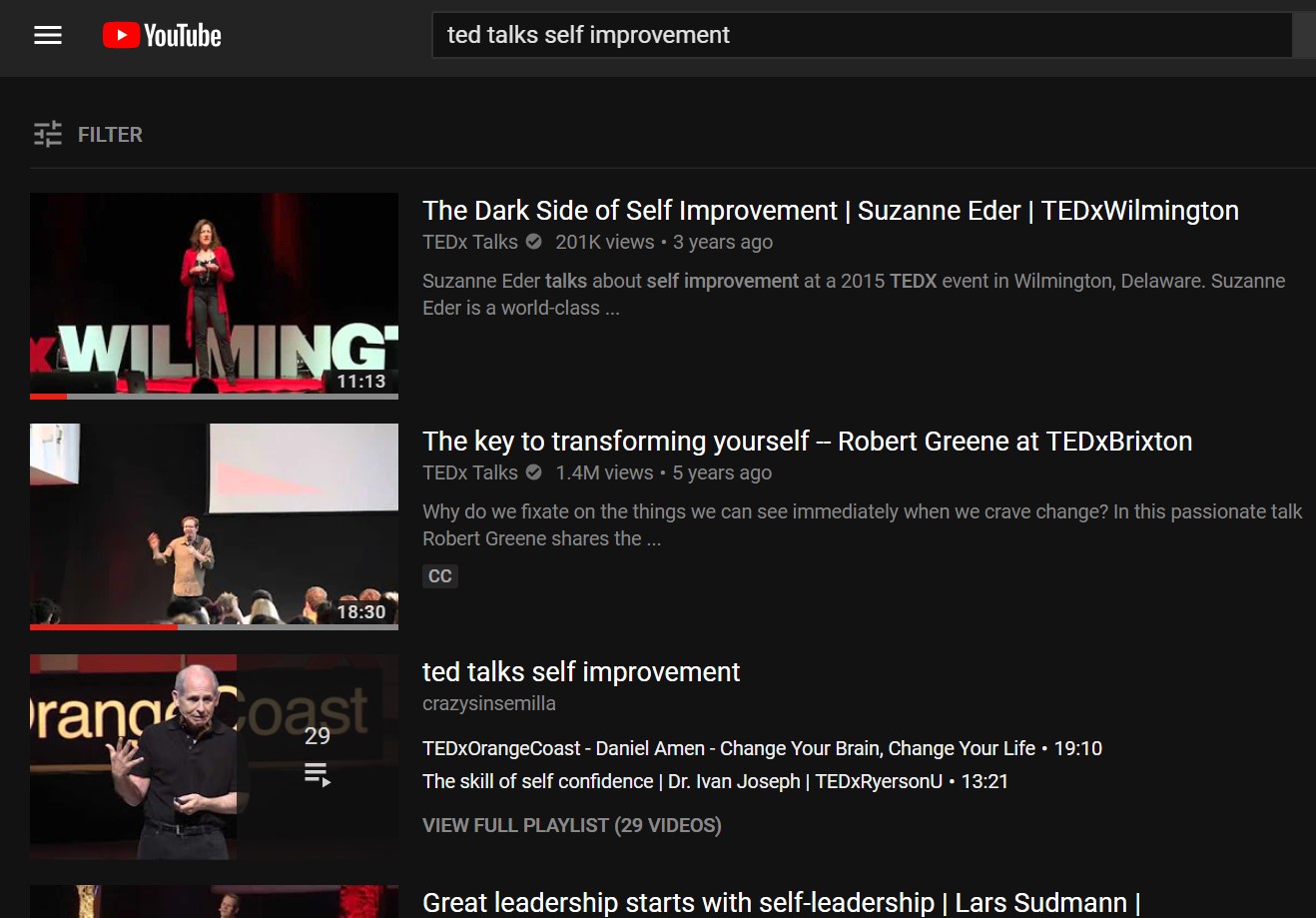This photo captures a YouTube search result page in landscape orientation. The background is predominantly black with a lighter gray header at the top, forming a rectangular gray box. On the left side of the header is a white hamburger menu icon, followed by YouTube's logo: a red rectangle with curved edges and a white play button in the center. Next to the logo, the word "YouTube" is displayed, and adjacent to it is a black search box with white text reading "TED Talks Self-Improvement."

Beneath the search box, there is a gray "Filter" option. A thin gray line runs below this area, demarcating the header from the search results. 

The first result features a woman speaking in a video titled "The Dark Side of Self-Improvement" by Suzanne Etter, which has a duration of 11 minutes and 13 seconds. The second result shows a man speaking in a video titled "The Key to Transforming Yourself" by Robert Greene, with a length of 18 minutes and 30 seconds. The third result displays a man in a black shirt among a collection of 29 other videos, and it is captioned “TED Talks Self-Improvement." There is an option to "View Full Playlist" next to this caption.

At the bottom of the photo, a partially visible video is titled "Great Leadership Starts with Self-Improvement" by Lars Sudman.